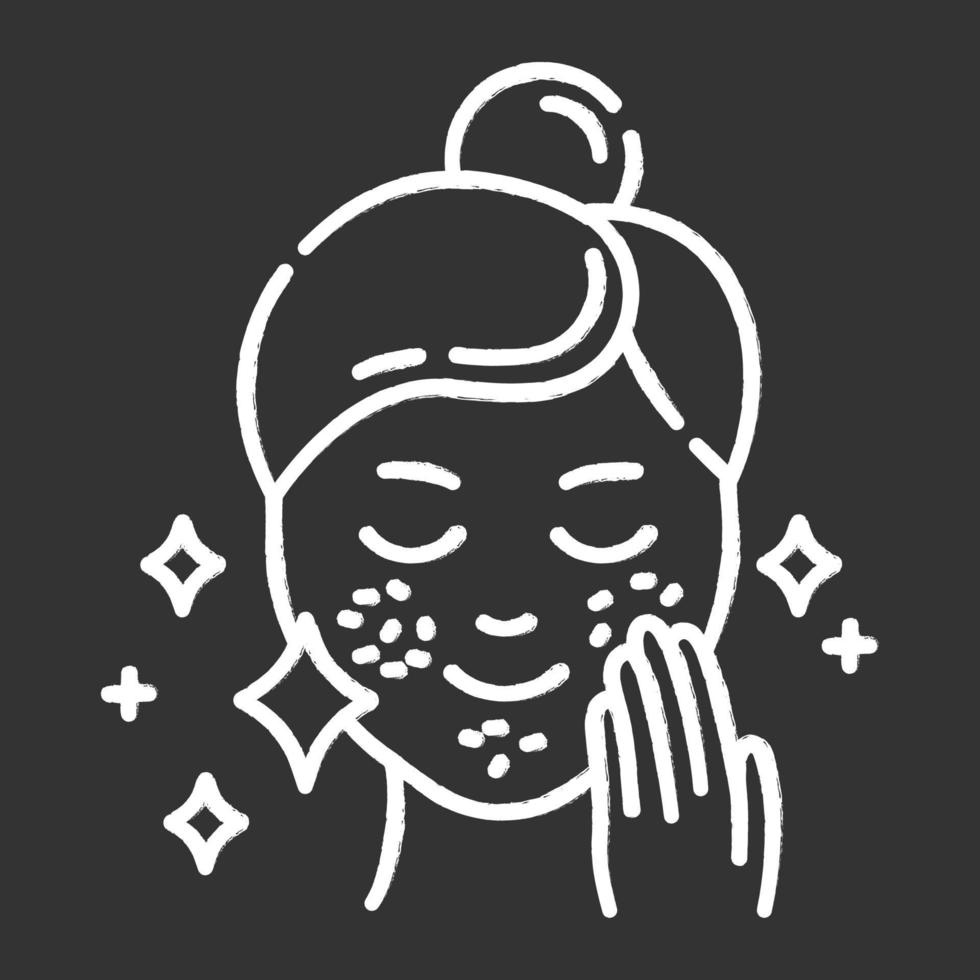This is a black-and-white, square-shaped digital illustration with a dark, almost black, background. In the center, there's a simple but textured line drawing of a young woman's face, created with thick, paint-like strokes that have uniform, rounded endings. Her hair is tied in a bun, and the drawing includes minimal yet expressive details. She has closed, slightly curved eyes created by two gentle lines each, dotted freckles on her cheeks, and a subtle, line-drawn smile. Her left hand is raised to her left cheek, and around her face are small decorative elements, including diamond shapes and plus symbols, which add a sense of sparkle and emotion to the image. It appears to convey a serene and affectionate mood.